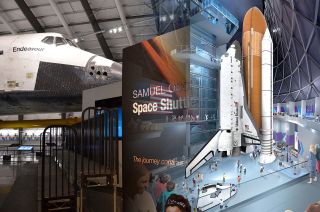The image depicts the interior of a NASA-related space museum, featuring a slotted metal ceiling and black and gray beams. Dominating the upper left corner is the Endeavor Space Shuttle, which is white with a black nose and the name “Endeavor” displayed in black letters. The shuttle is mounted from the ceiling, appearing to dangle in mid-air. Beneath the shuttle, there are small black gates with rounded tops. Central to the image and slightly to the right is a prominent billboard with partially readable text, "Samuel something Space Shuttle," showing images of rockets and people; the images on the billboard include a large space shuttle, akin to the one hanging, positioned vertically as though on a launch pad with associated brown and white rockets. To the right of this billboard, another illustration also depicts rockets and space shuttles, providing additional context to the main exhibit. The lower portion of the image includes seating benches, and a hint of what appears to be the top of someone's head can be seen in the bottom right corner. The overall atmosphere is that of an educational and informative exhibit area, dedicated to showcasing NASA’s space exploration achievements.